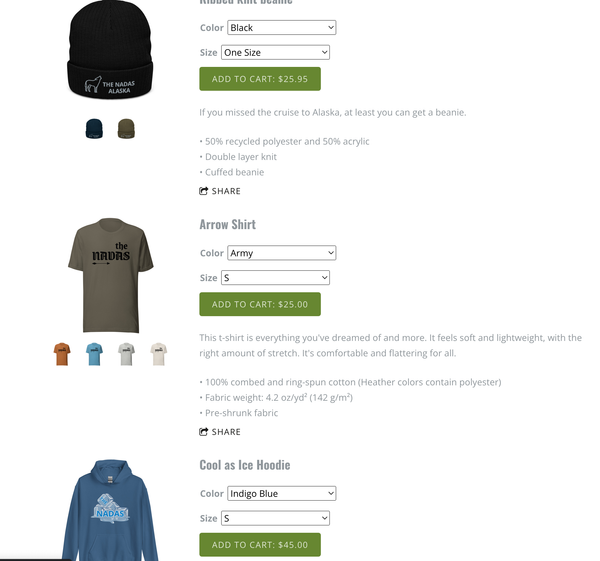This website showcases a selection of Nadas, Alaska-themed clothing items neatly organized into distinct sections. Each section features a product image, a dropdown menu for color and size options, an add-to-cart button, and a detailed description of the item.

At the top of the page is a classic beanie featuring a cow logo and the text "Nadas, Alaska." This beanie is available in two color options: black and dark green.

Directly below the beanie, there is a stylish green shirt with the word "Nadas" emblazoned across the front in an old English font. This shirt is offered in multiple colors, including orange, light blue, light gray, and white, with size options clearly accessible via the dropdown menu.

Further down the page, another beanie is presented, this time in blue and adorned with a graphical picture accompanied by the text "Nadas" in blue. The beanie itself is blue and comes in two additional colors: black and very dark green.

Each item is meticulously detailed to provide a comprehensive view of the available selections, ensuring a smooth and informed shopping experience for potential customers.